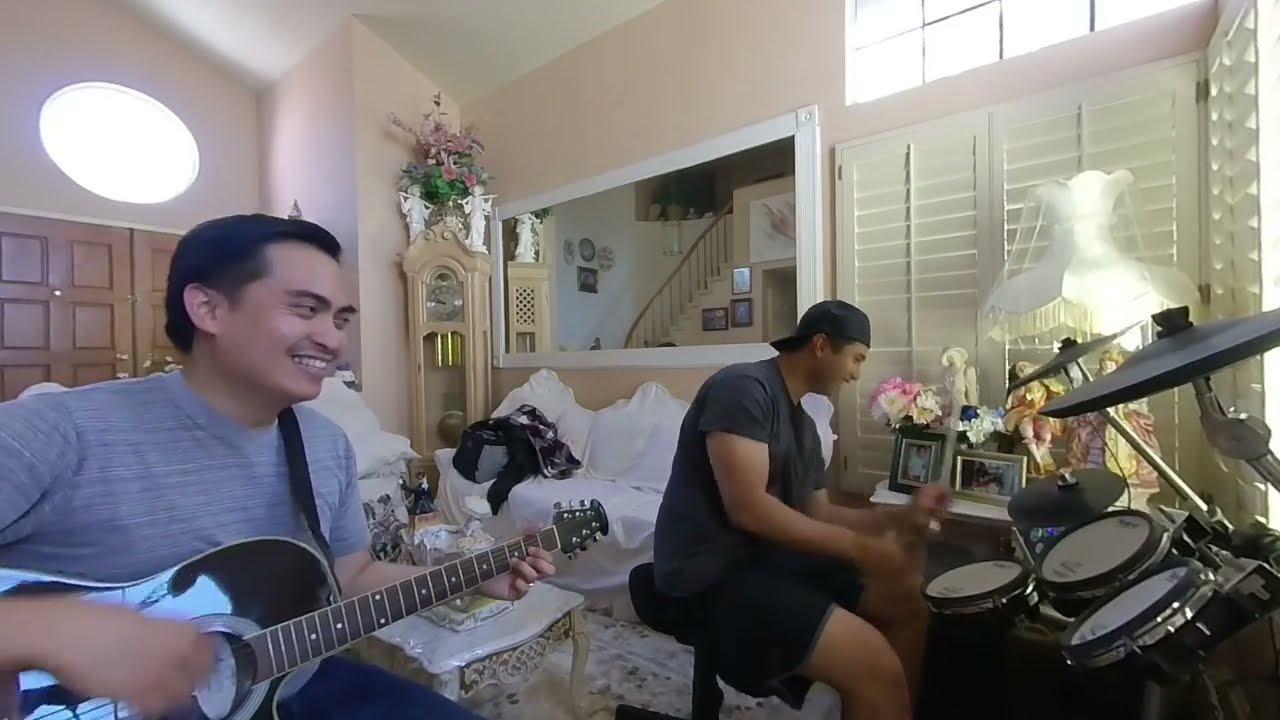The image depicts two smiling, excited men playing music inside a living room characterized by old-school decor with lots of curves on the furniture and a frilly aesthetic, including pink walls and floral elements. The man on the left, wearing a subtly striped gray t-shirt and blue pants, has short black hair and is playing a wooden guitar while smiling towards the other man. The man on the right, dressed in a dark gray t-shirt, black shorts, and a backwards black baseball cap, is playing the drums, with his blurred hands indicating motion. In the background, you can see double wooden doors on the left side with an oval window above them letting in bright light. On the right side, there is a rectangular window with thick white wooden blinds. Additional background details include a couch draped in cloth, a bag, a shirt, family photos, a clock adorned with tiny statues or sculptures, and a large bouquet of flowers. Both men appear to be of Asian descent, and the overall ambiance of the room suggests a homely and vibrant setting.